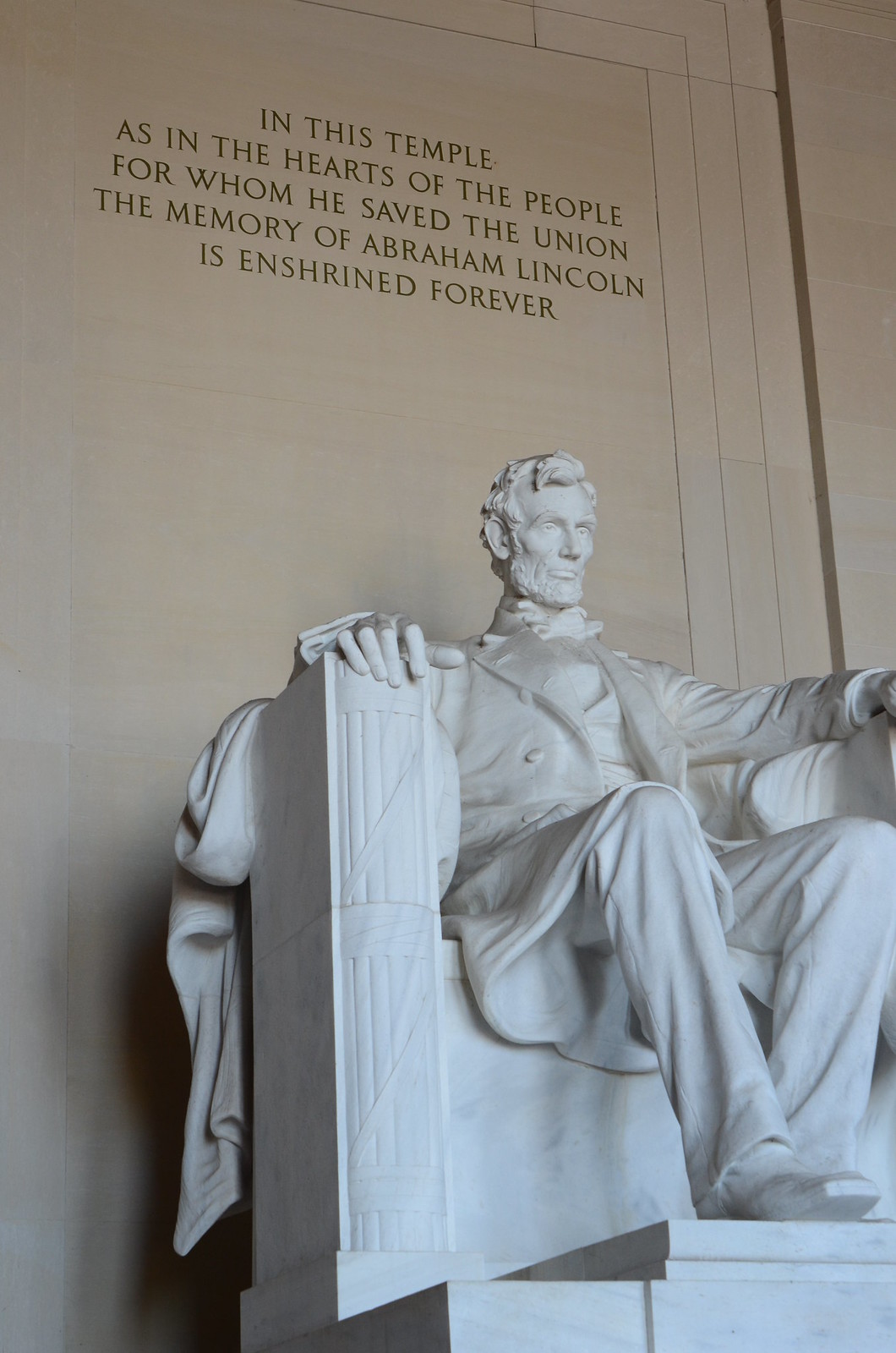This image captures the grandeur of the Lincoln Memorial, focusing on the iconic white marble statue of President Abraham Lincoln seated in a grand chair. The photo is taken from the lower right segment of the memorial, providing a detailed perspective of the statue's intricate details. Lincoln is sculpted with a beard, short hair, and dressed in a button-up jacket, long pants, and boots, with his hands resting on the side railings of the imposing stone chair. Drapery carved in stone hangs over the back of the chair, adding to the sculpture's intricate craftsmanship. Above Lincoln, etched into the whitish-tannish marble wall, is the famous inscription: "In this temple, as in the hearts of the people for whom he saved the Union, the memory of Abraham Lincoln is enshrined forever." The photograph is taken in daylight, highlighting the statue's imposing presence without the need for additional lighting, and capturing the timeless reverence of this historic monument.